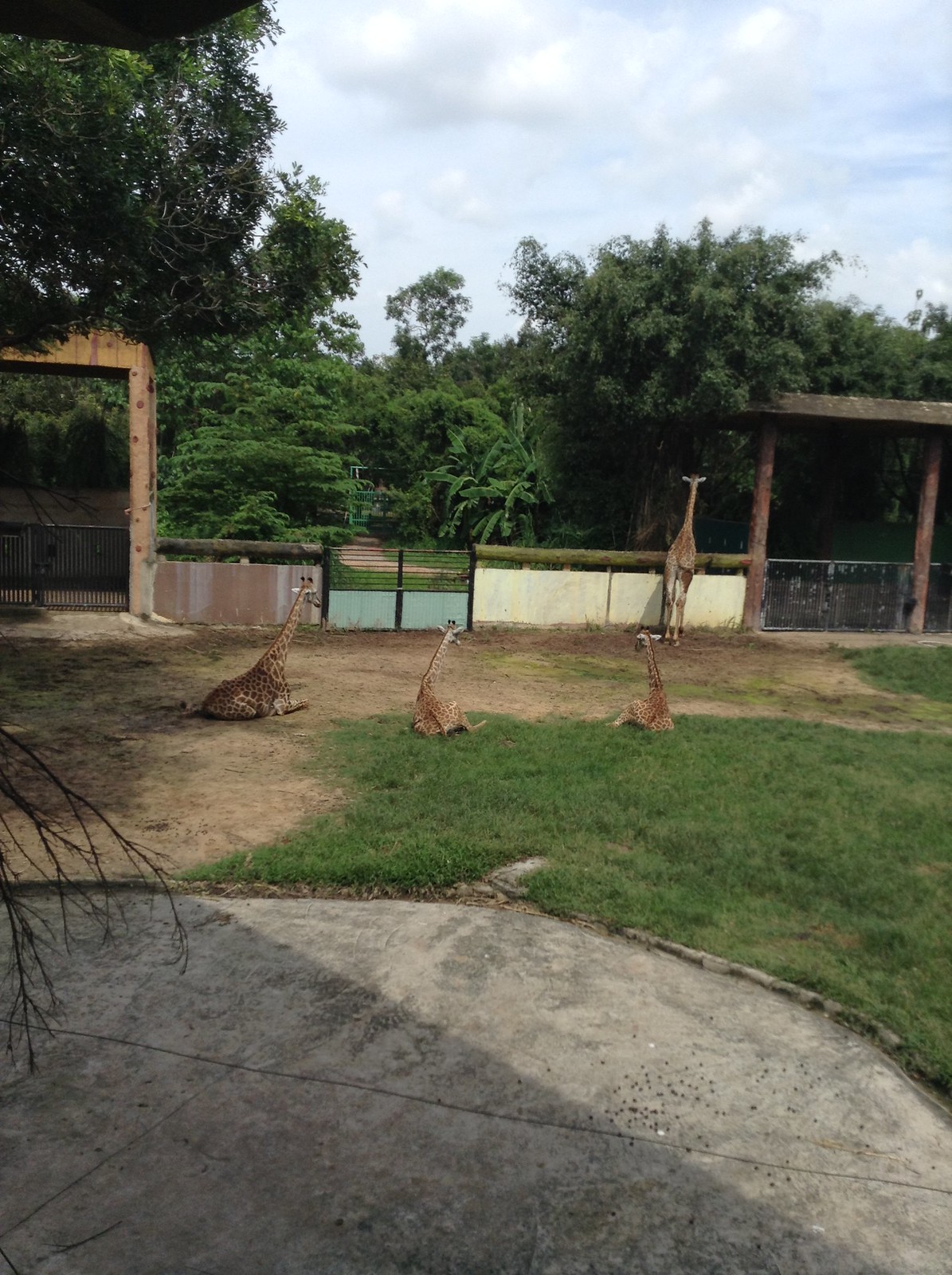The image depicts a zoo enclosure housing four giraffes. The enclosure's ground is a mix of dirt, grass, and a cement pad in the foreground. A tall wooden archway towers above the giraffes, with a partly see-through fence featuring black railings and a combination of blue and white materials at the bottom, alongside a striped brown section.

In the scene, one giraffe stands upright on all four legs, gazing over the wall in the distance, while three others are seated on the ground with their necks elevated, two resting on grassy patches and one on the dirt. All giraffes have their backs to the camera. Beyond the enclosure, the background showcases a variety of trees, including oaks and palms, under a sky with hazy clouds. A brown road runs along the periphery of the enclosure.